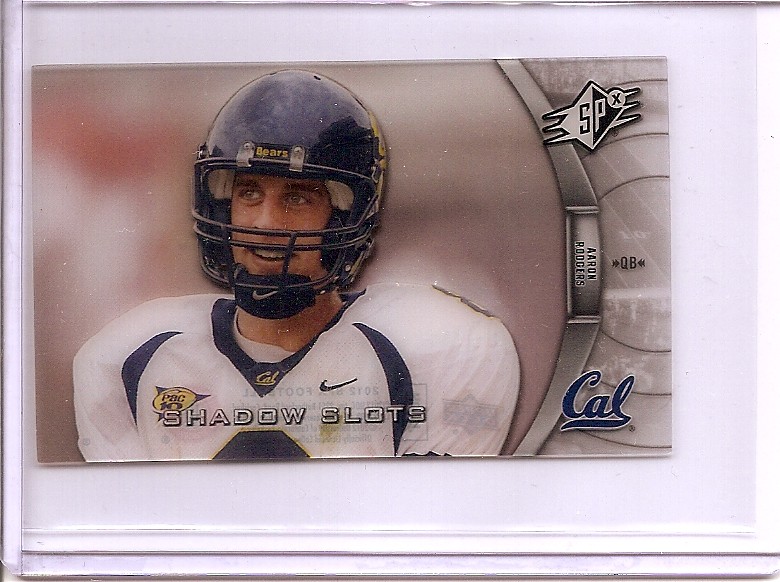This image features a detailed, collectible football card prominently displayed against a white background. The card, slightly diagonal and encased in a plastic protective sleeve, showcases a stylized drawing of Aaron Rodgers in the center. Rodgers is depicted in a dark blue helmet with a black face guard and a distinctive Nike chin strap, which features a yellow Nike Swoosh. He is dressed in a white jersey adorned with blue slants on the shoulders and a blue Nike Swoosh on the right shoulder pad. Rodgers is looking off to his right with a slight smile on his face. The neckline of his jersey is dark blue with "Cal" printed in gold, and there's a subtle drawing of a football to the left of this print. 

Text elements are prominently displayed across the card. At the bottom, in raised white lettering, it reads "shadow slots." The lower right corner features "Cal" in blue script. The upper right corner contains a logo with the letters "SP" and an "X" in the upper right corner of the logo. Additionally, "Aaron Rodgers QB" is written in a banner. The card's color scheme includes gray, white, dark blue, purple, yellow, and black, enhancing its collectible appeal. The background is blurred, focusing attention on the central image. The card appears to be of special edition, indicated by its slight thickness and the use of a protective sleeve for preservation.